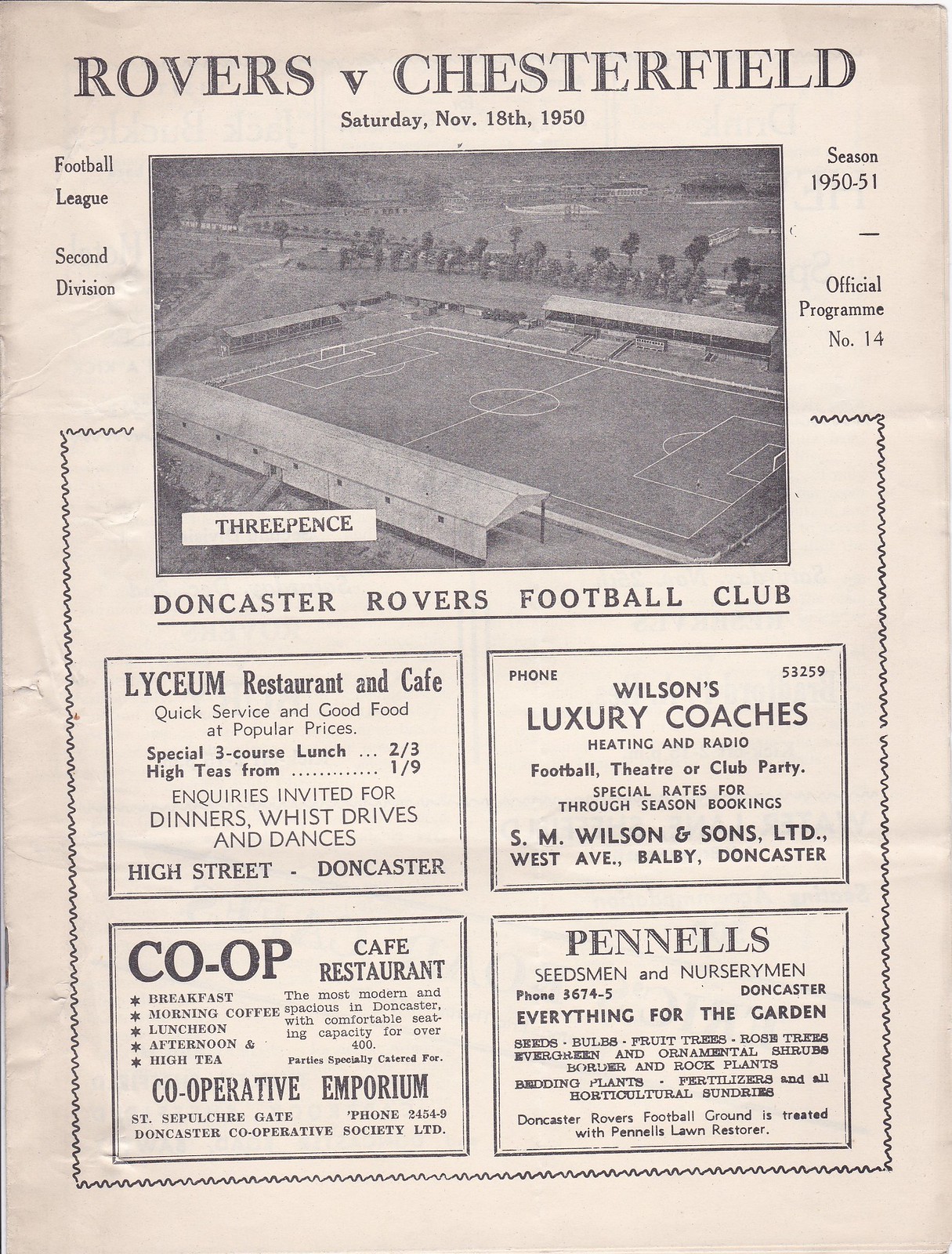This vintage advertisement poster from an old sports event showcases an aged cream-colored paper with slightly wrinkled and brown edges, indicating its historical value. At the top, the poster announces "Rovers vs. Chesterfield, Saturday, November 18, 1950," in bold black text. The center features a slightly blurry, black-and-white photograph of a football (soccer) field taken from an elevated viewpoint. To the left of the photograph, the text reads "Football League, 2nd Division," while the right side states "Season 1950-51, Official Program No. 14." Just below the image, in black lettering, is "Doncaster Rovers Football Club." The bottom section of the poster contains four rectangular advertisements highlighting various sponsors: the Lyceum Restaurant and Cafe, Wilson's Luxury Coaches, Pennell's Seedsmen and Nurserymen, and Co-op Cafe Restaurant. The poster also mentions "three pence" as the price for the program.